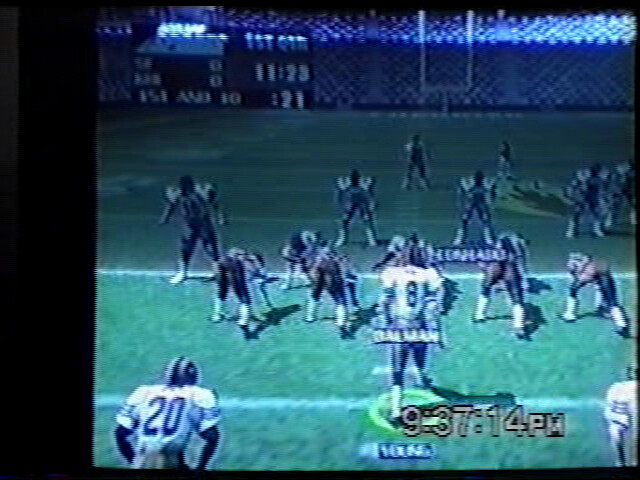This image is a close-up photograph of a television screen displaying an old-school, pixelated NFL video game. The scene depicts a football game with the Dallas Cowboys, distinguishable by their white and blue uniforms. The central figure is a quarterback in a white jersey with gray pants, bearing the number 8, likely representing Troy Aikman. Behind him are two more Dallas offensive players, the tops of their jerseys barely visible. Across from them, players of the opposing team face the viewer.

The green football field features white stripes, and near the upper edge, a white goalpost is visible. The background showcases blue, pixelated stands, representing the crowd. The upper left corner of the screen displays a digital scoreboard, reading "0 - 0" with a game clock showing "11:23" and "21" underneath. In the bottom right corner, there's another time display reading "9:37 :14 PM" in a yellow or tan color, with some other unreadable text below it. The entire scene has a blue tint, further emphasizing the game's retro aesthetic.